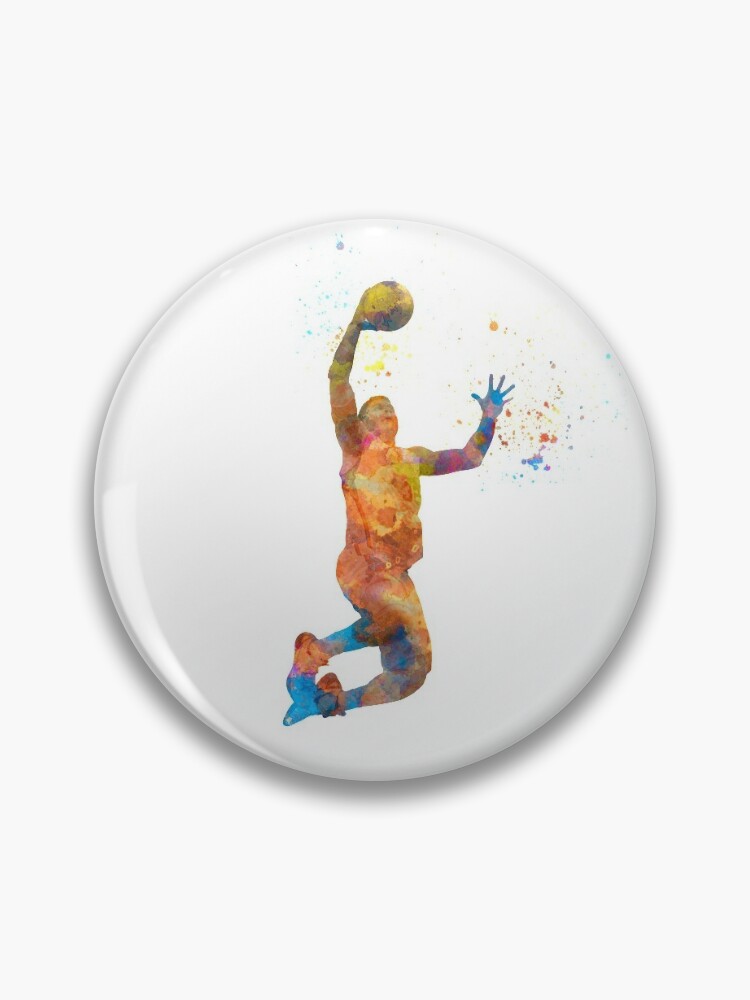The image features an artistic piece presented on a glossy, circular white object, resembling a button or a plate. The object showcases a vivid illustration of a male basketball player mid-air, seemingly about to dunk a basketball with his right hand outstretched. The player, donned in a basketball outfit including a jersey with the number three, shorts, and sneakers, is depicted in a dynamic pose with bent knees, looking towards the top right where he is leaping.

The artwork employs a vibrant, multicolored palette with hues of orange, yellow, blue, red, pink, brown, and purple, giving the player a watercolor or chalk-like texture. Surrounding the player's arms, there are artistic splatters of paint, enhancing the dynamic and visually arresting quality of the piece. The entire artwork is set against a white background, both on the circular object and the surrounding area, emphasizing the striking contrasts and lively colors of the design.